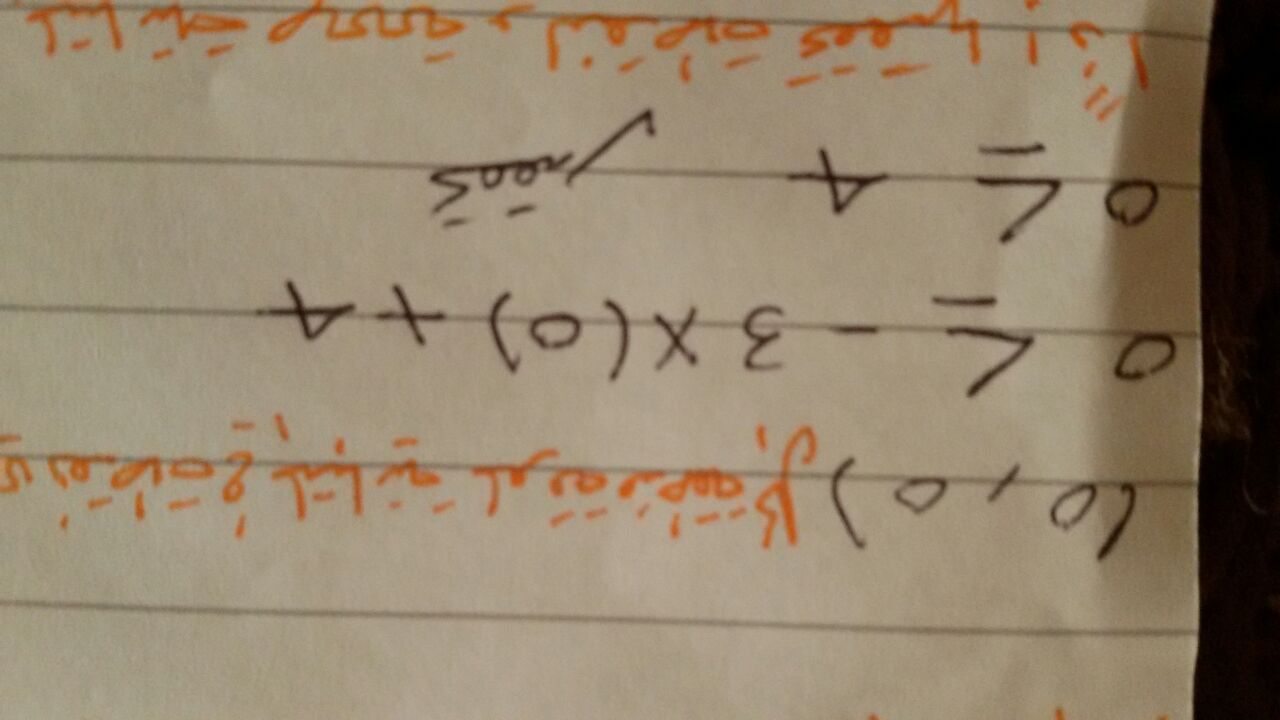An upside-down photograph showcases a piece of white paper lined with gray horizontal lines. The paper is marked with intricately detailed inscriptions in both black and orange ink, which appear to be mathematical equations and annotations. 

The first line features numbers and symbols written in black, including a segment with parentheses, zeros, and slashes ("(0/0)"). To the right of this, there is additional complex writing in orange pen.

Beneath this, a second line presents another mathematical expression in black ink: "0 ≤ -3(0 + 4)". Followed by this, the third line states, "0 ≤ 4," in black ink.

The final line at the bottom of the paper is entirely inscribed in orange ink, consisting of intricate and possibly unintelligible text that appears either as further mathematical notation or an undecipherable script. This line predominantly resembles squiggly shapes, making it difficult to ascertain whether it represents math or another form of notation.

Overall, the document contains four lines of written content: the first and fourth in both black and orange, and the second and third exclusively in black.